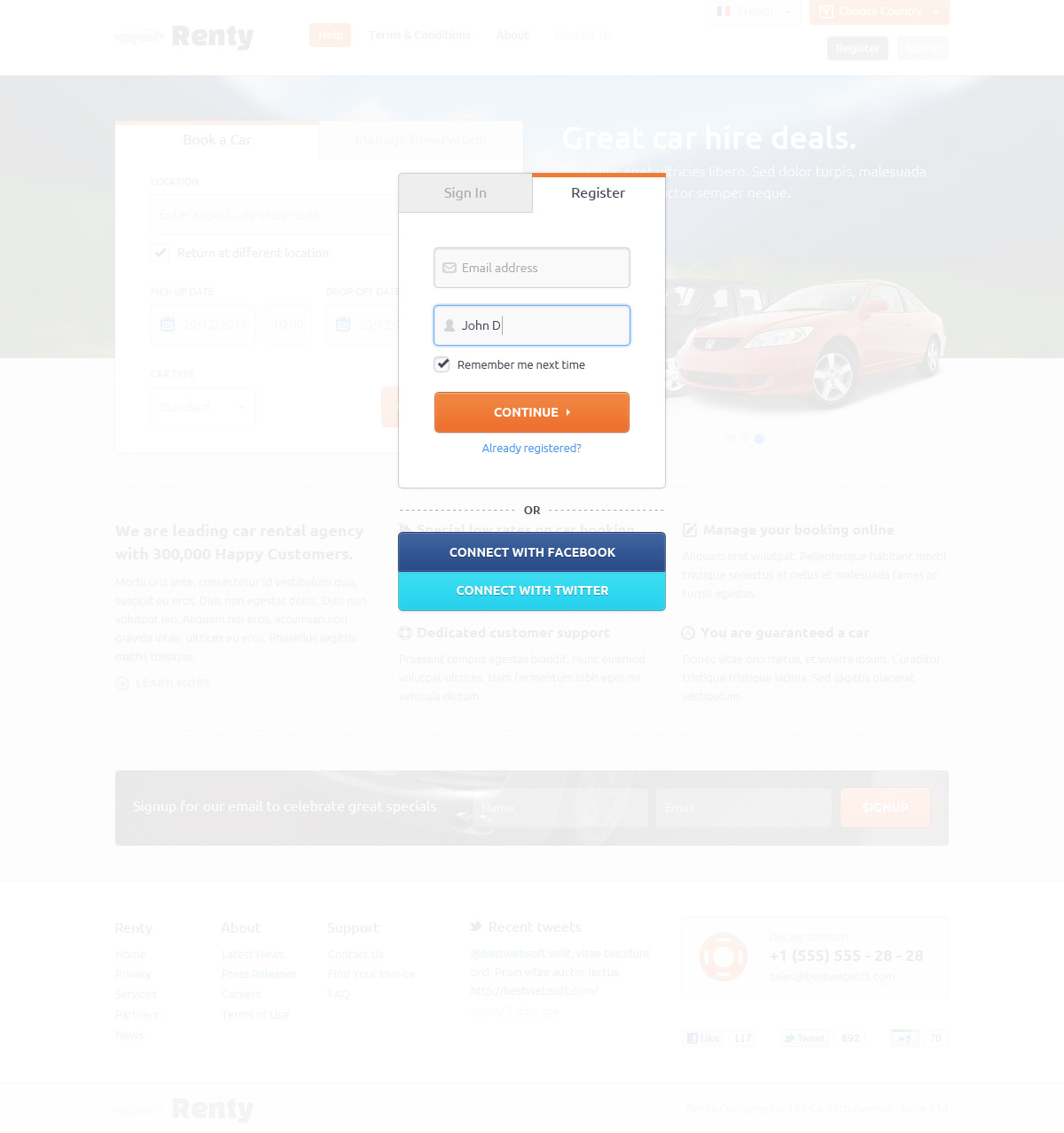The image depicts a webpage designed for user authentication, featuring a blurred background. Centrally located on the page is a white box dedicated to sign-in and registration functionalities. Within this box, the "Sign In" option is positioned at the upper left corner, encased in a grey box. Adjacent to it, against the white background, is the "Register" option in black text.

An orange outline accentuates the upper portion of the white box, extending from the center to the right edge. Below the "Sign In" section, there are input fields for email address and name. A checkbox labeled "Remember me next time" is also present. Below these fields, an orange "Continue" button is prominently displayed.

Further down, a blue link prompts users with "Already registered?" Additionally, options to connect via social media are provided, with dark blue "Connect with Facebook" and light blue "Connect with Twitter" buttons, both featuring white text.

In the blurred background, a red car is discernible in the upper right corner, accompanied by the text "Great car hire deals" above it. The rest of the text is unreadable. At the very top of the page, the site name "Renty" (spelled r-e-n-t-y) is visible on the upper left side. The bottom of the page contains more text and information, which is also blurred and unreadable.